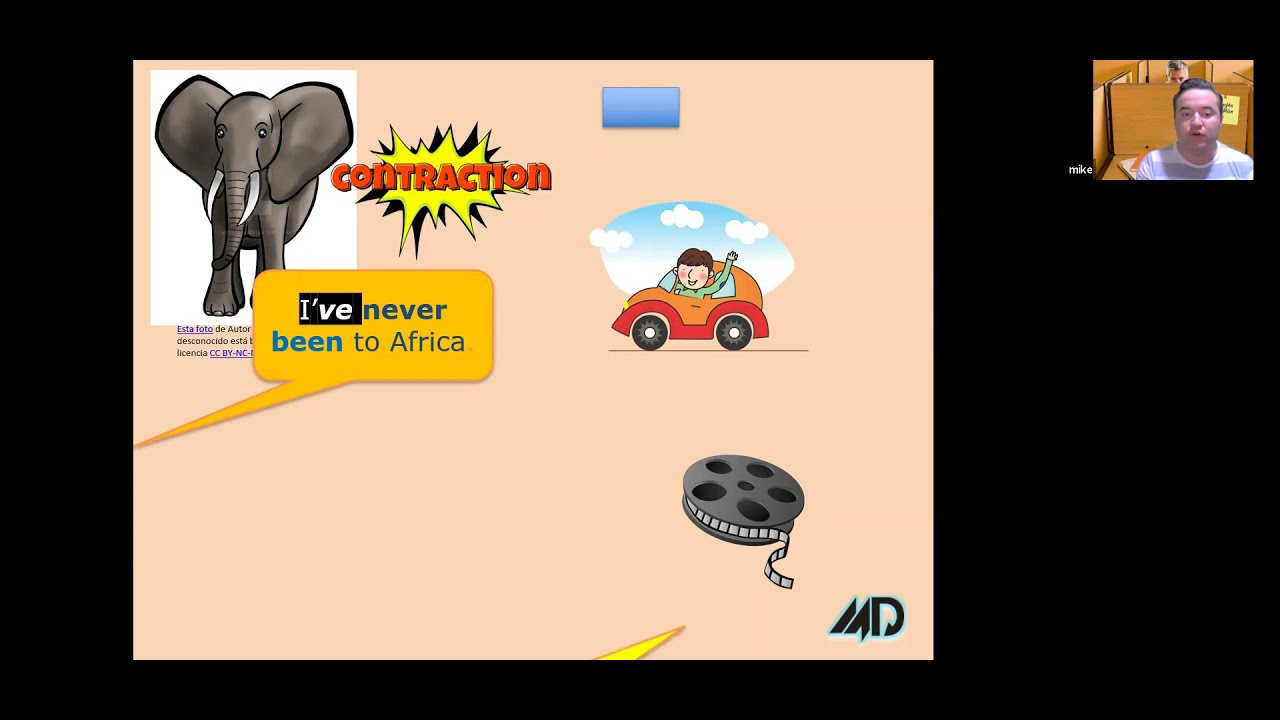This image appears to be a screenshot from an online teaching program focusing on contractions. The main slide has a peach-colored background occupying about two-thirds of the screen. On the left side, there is clip art of an elephant next to a yellow explosive "bam" sign with the word "contraction" written in red. Below this, a mustard-yellow speech bubble with a black background features the text in white: "I've never been to Africa."

To the right of the speech bubble, there is clip art of a red convertible car with a cloud behind it, driven by a person with an outstretched hand and a long sleeve shirt. Above this car is a blue rectangle, and below it is an old-fashioned film reel with "MD" written in the bottom right corner.

In the top right corner of the slide, there is a small photo of a man who appears to be the teacher, possibly named Mike. This photograph contributes a real-life element to the otherwise illustrated and stylized slide, which seems to depict a lesson on contractions within a virtual classroom setting.